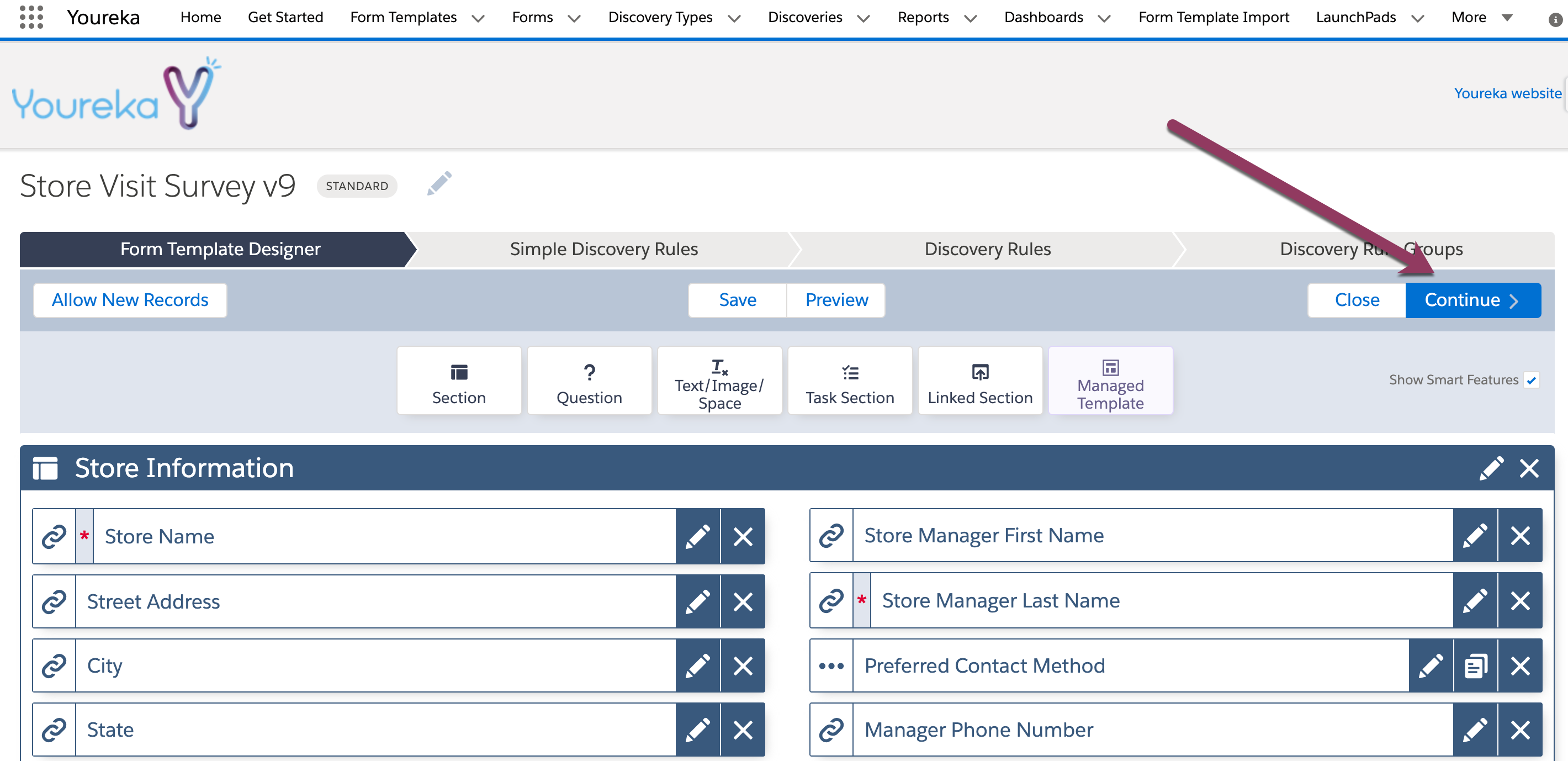**Descriptive Caption:**

This image is a cropped screenshot of the Eureka webpage that focuses on various interface elements. At the very top of the screenshot, there is a small white banner displaying the word "Eureka" on the left side. To the right of "Eureka," a row of navigation options is visible, each accompanied by a drop-down box: Home, Get Started, Form Templates, Forms, Discovery Types, Discoveries, Reports, Dashboards, Form Template Import, Launchpads, and more.

Beneath this, a gray header is visible, featuring the Eureka logo on the left. On the right side of this header, "Eureka website" is written in small blue, hyperlinked text. Below this gray header, there is a white bar which starts with the text "Store Visit Summary V9" on the left side. Adjacent to this text is a gray button labeled "Standard," accompanied by a pen icon that allows for title editing.

The main content below these navigation elements includes several options such as Form Template Designer, Simple Discovery Rules, and Discovery Rule Groups. The "Form Template Designer" option is currently selected. Additionally, a red arrow has been digitally added to the screenshot, pointing to a "Continue" button on the right side of the page. This arrow and the highlighted selection demonstrate the process of navigating to the Form Template Designer, entering store information into the designated text boxes, and then pressing "Continue" to proceed.